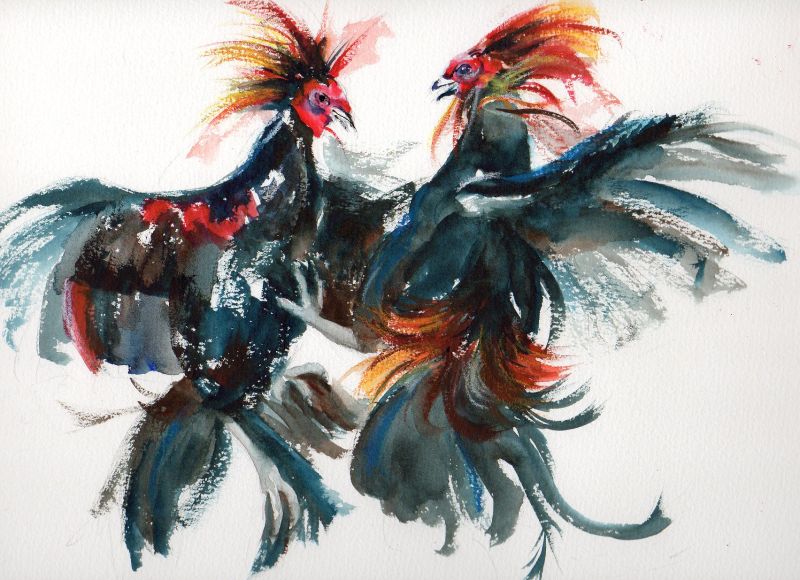This engaging watercolor illustration features two vividly colored roosters, possibly bantams, facing each other against a stark white background. Their vibrant heads, primarily red, are framed by a mix of yellow, red, and darker feathers. The rooster on the left showcases more red, contrasted by darker body feathers, while the rooster on the right displays a darker top with striking orangey-red hues partway down. Both roosters have their wings dramatically spread out behind them and their mouths open, perhaps arguing, creating an impression of impending confrontation. Their tail feathers dangle below them, adding to the dynamic and somewhat abstract composition. Despite the suggestion of a fight, with claws raised and wings poised, the overall scene appears more evocative of heightened tension rather than explicit violence. Their beaks are subtly white, outlined in black, anchoring the intricate play of colors on their animated faces and bodies.